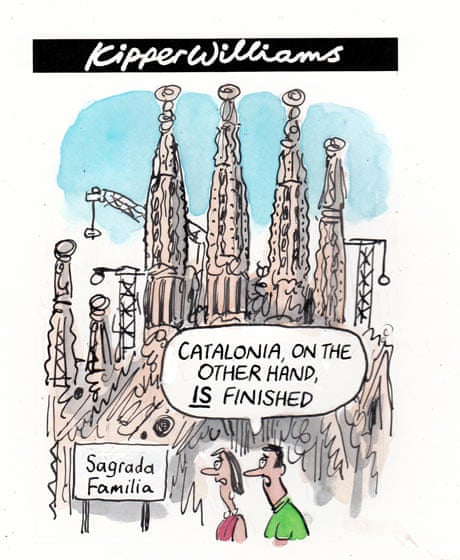The cartoon by Kipper Williams depicts a couple, a heavyset man in a green shirt and a woman in a pink shirt, walking towards the left in front of the iconic Sagrada Familia in Spain. The backdrop features the unfinished basilica, surrounded by cranes, emphasizing ongoing construction against a light blue sky. The sign in the background reads "Sagrada Familia," and the man comments humorously, "Catalona, on the other hand, is finished," potentially alluding to differing viewpoints on Spanish politics or infrastructure. The overall tone suggests a satirical take on the complexities of Spanish societal themes, with industrial elements framing the scenario. A black bar at the top with the label "Kipper Williams" marks this scene as one of his political cartoons.